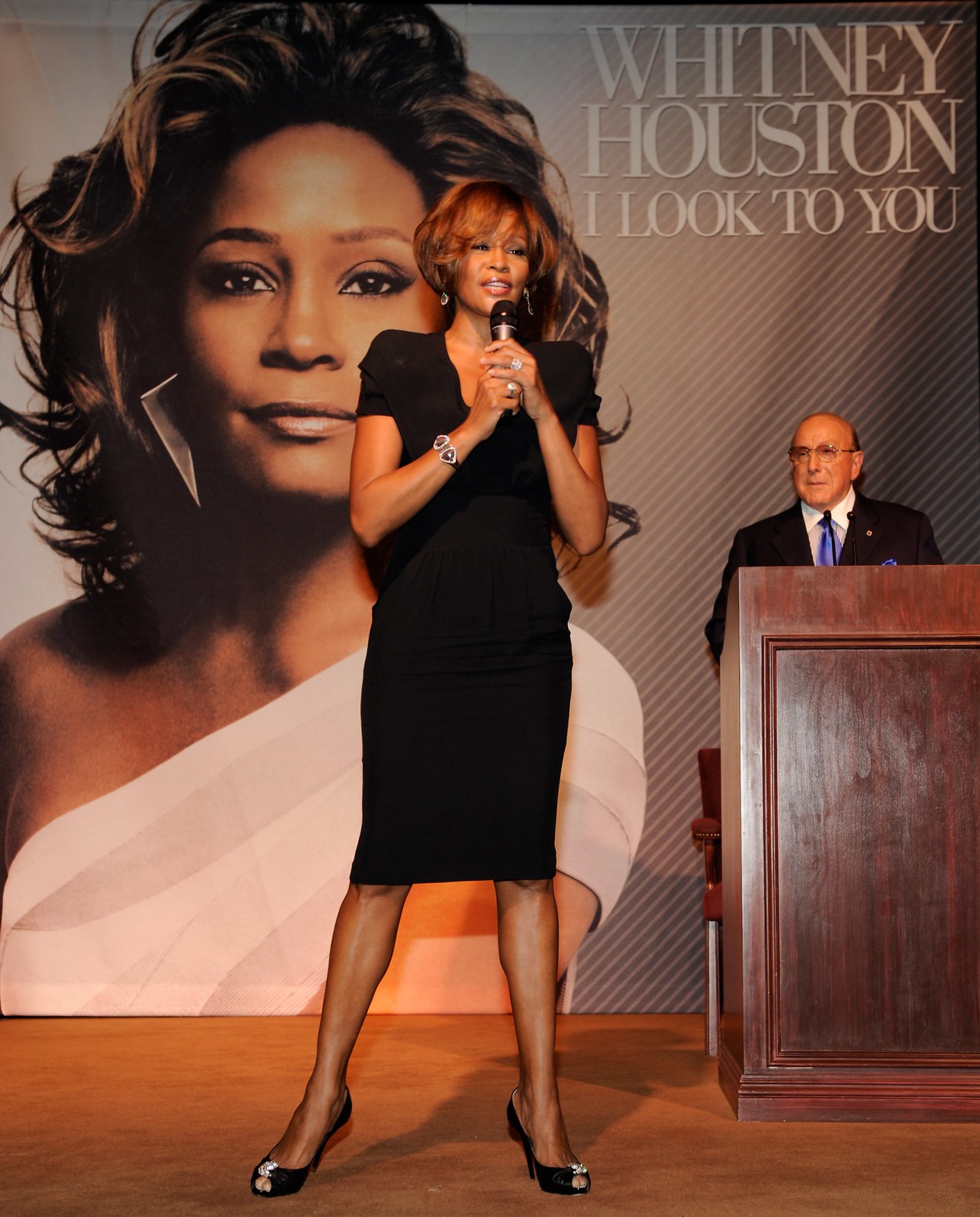This photograph captures Whitney Houston standing on a stage, holding a microphone with both hands near her mouth. She is adorned in a short, elegant, black dress and high-heeled shoes, accentuated by a bracelet and multiple rings. Positioned to her right is an older, balding gentleman clad in a dark suit with a white shirt and a royal blue tie, standing behind a dark wooden podium. 

The background is dominated by a large banner featuring a picture of Whitney Houston in a white dress. In the upper right corner of the banner, the text reads "Whitney Houston: I Look to You," suggesting a possible promotion of a book or an album. Notably, there is also a hint of a chair peeking out from the left side of the podium. Whitney appears to be addressing the audience, emphasizing her role as a speaker rather than a singer in this moment.